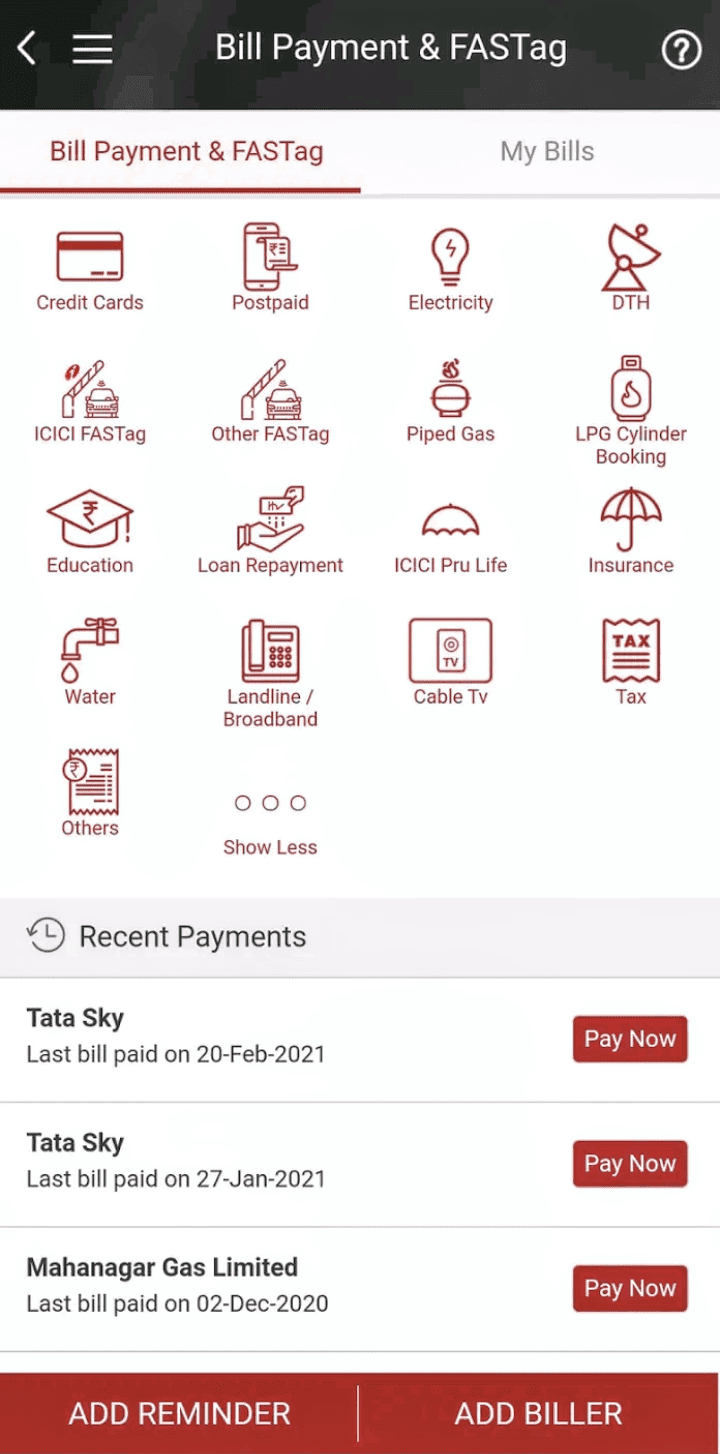Here is a refined and detailed caption:

---

A smartphone screenshot showcasing a bill payment application is visible. The top section features a black header with a back arrow on the left, a hamburger menu on the right, and centered text that reads "Bill Payment and FASTAG," with "FASTAG" dynamically displayed as "F-A-S-T" in uppercase letters followed by lowercase "ag" and a question mark in a white circle on the far-right.

Beneath this header, the interface displays a distinct red and white theme, with black accents. There's a prominent red underline beneath the "Bill Payment and FASTAG" text indicating it is the selected tab, while the text "My Bills" appears to the right in gray.

The main body of the screen is divided into several lines of icons categorizing the various bill payment options:
- First row: Credit Cards, Postpaid, Electricity, and DTH.
- Second row: ICICI FASTAG, Other FASTAG, Pipe Gas, and LPG Cylinder Booking.
- Third row: Educational Repayment, ICICI Prudential Life, and Insurance.
- Fourth row: Water, Landline, Broadband, Cable TV, and Tax.
- Fifth row: Others and Show Less.

Below the icons, there's a section for recent payments. It lists:
1. Tata Sky, with the last bill paid on February 20th, 2021, and a red "Pay Now" button.
2. Another entry for Tata Sky, with the last bill paid on January 27th, 2021, accompanied by a "Pay Now" button.
3. Maha Nadjar Gas Limited, with the last bill paid on December 2nd, 2020, also featuring a "Pay Now" button.

At the bottom of the screen are two buttons. The one on the left is red with white text saying "Add Reminder," and the one on the right is white with red text saying "Add Biller."

---